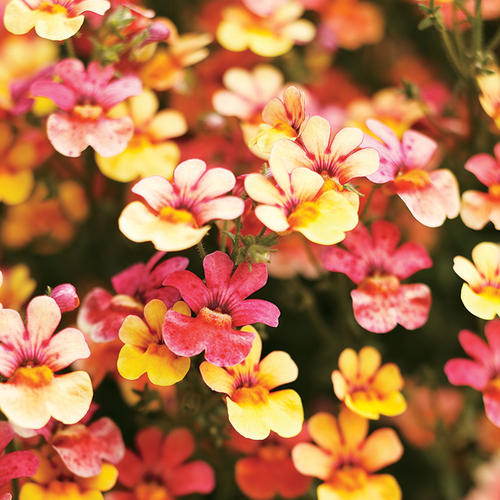This close-up photograph captures an intricately detailed view of a flowering bush, with small, vibrant flowers grouped closely together on their green stems. Each flower, reminiscent in size to a buttercup but slightly larger, boasts a diverse palette of saturated colors, including vivid reds, yellows, and creams. The petals, numbering five per flower, often show blended hues of pink, red, and yellow at their centers. While the foreground flowers are in sharp focus, richly displaying their detailed petals and colorful centers, the background gradually blurs, showing a softer amalgamation of colors and some unopened buds that appear as green nubs. The overall scene is accented by lush green foliage interspersed among the flowers. Some flowers in the background exhibit darker red splotches, resembling tie-dye patterns, adding to the visual complexity and beauty of the image. The sunlight casts a gentle haze around some petals, enhancing the ethereal quality of the photograph.